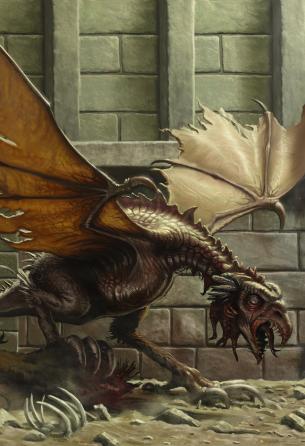This digital illustration depicts an imposing, snarling dragon standing on its hind legs in what appears to be the basement of a stone castle. The background features a stone wall partially concealing a bricked-up window, adding to the dungeon-like atmosphere. The dirt and rock floor is littered with old, unidentifiable bones, including remnants of ribcages, suggesting the dragon’s previous feasts. The dragon itself is a terrifying, skinny figure, seemingly carved out of copper, with wings extended slightly upward displaying a brownish-orange tint and signs of damage. Its face is dominated by a gaping mouth, visible tongue, and thick, wrinkled brow, emphasizing its menacing appearance as it looks down, poised to attack. The overall image is dark, dominated by greys, enhancing the foreboding and sinister mood.